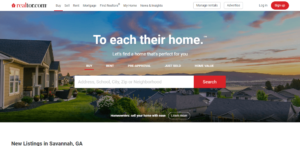This image depicts a promotional banner from an unidentified house listing website, albeit blurred and small in size. The banner prominently displays a tagline reading, "To each their own, to each their home," signifying a personalized approach to home searching. In the upper right corner, there is a red button, likely designated for user login or registration, although the text is indistinct.

The centerpiece of the banner features a scenic image of suburban houses bathed in the warm hues of a sunset, with clouds scattered across the sky and a grassy foreground adding to the idyllic setting. Dominating the middle of this picturesque scene is a search box with a conspicuous red search button, inviting users to start their home search.

At the bottom of the banner, clearly readable text announces "New listings in Savannah, Georgia," suggesting a focus on current property offerings in that area. The top portion of the banner includes various navigation tabs and additional clickable options located just above the search box, though the exact text remains unclear due to the image's blurriness. Overall, the banner aims to engage potential homebuyers with its inviting imagery and essential search functionality.